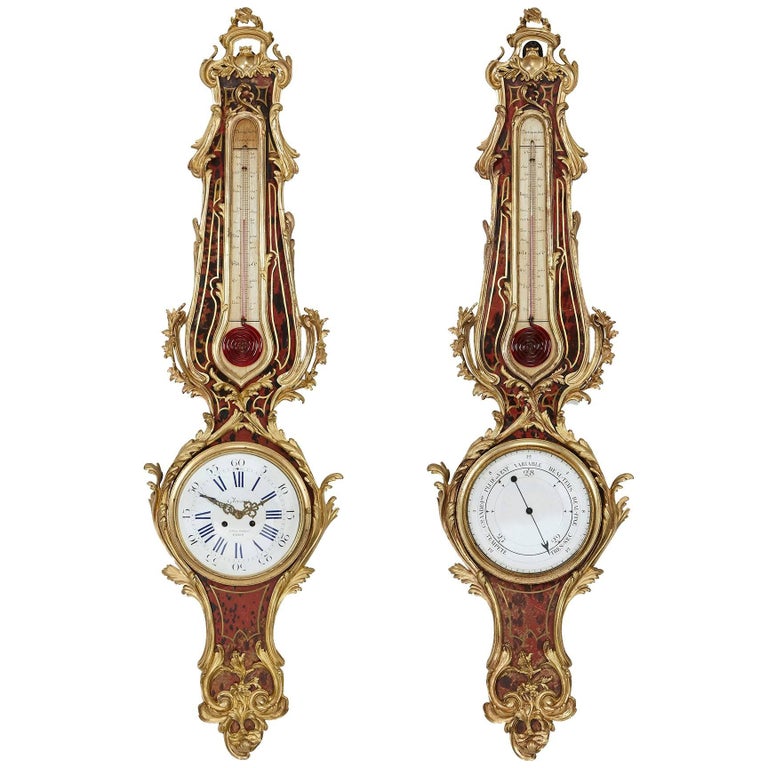The image showcases two intricately designed gold watches, exuding an air of elegance and luxury. Both watches are adorned with ornate details, featuring delicate designs resembling plants or leaves intertwined around the circular faces of the timepieces. On the left side of the image is a traditional wristwatch, while the right side appears to display an instrument that resembles a weather barometer, although its exact purpose is unclear. The craftsmanship of both pieces highlights their refined and sophisticated aesthetic.